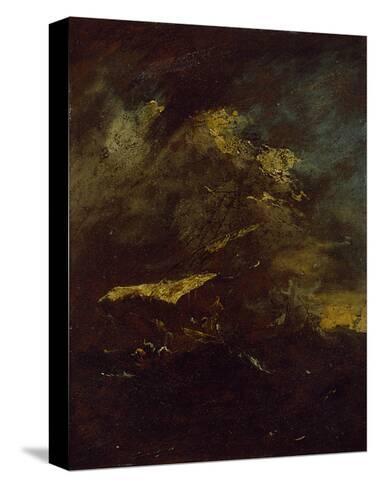The image depicts a dark and gloomy painting propped upright, possibly leaning slightly to the right. The scene within the painting conveys a tumultuous ocean during a storm, with monstrous, dark grayish-yellow waves crashing violently against each other. The sky adds to the ominous atmosphere, streaked with colors ranging from navy blue to brown and yellow. The dark hues dominate the overall composition, making it difficult to distinctly identify specifics in the image. The painting is framed in black and casts a subtle shadow on the bottom left, suggesting that the light source is coming from the front right. The white background of the scene accentuates the painting's dark, stormy character.